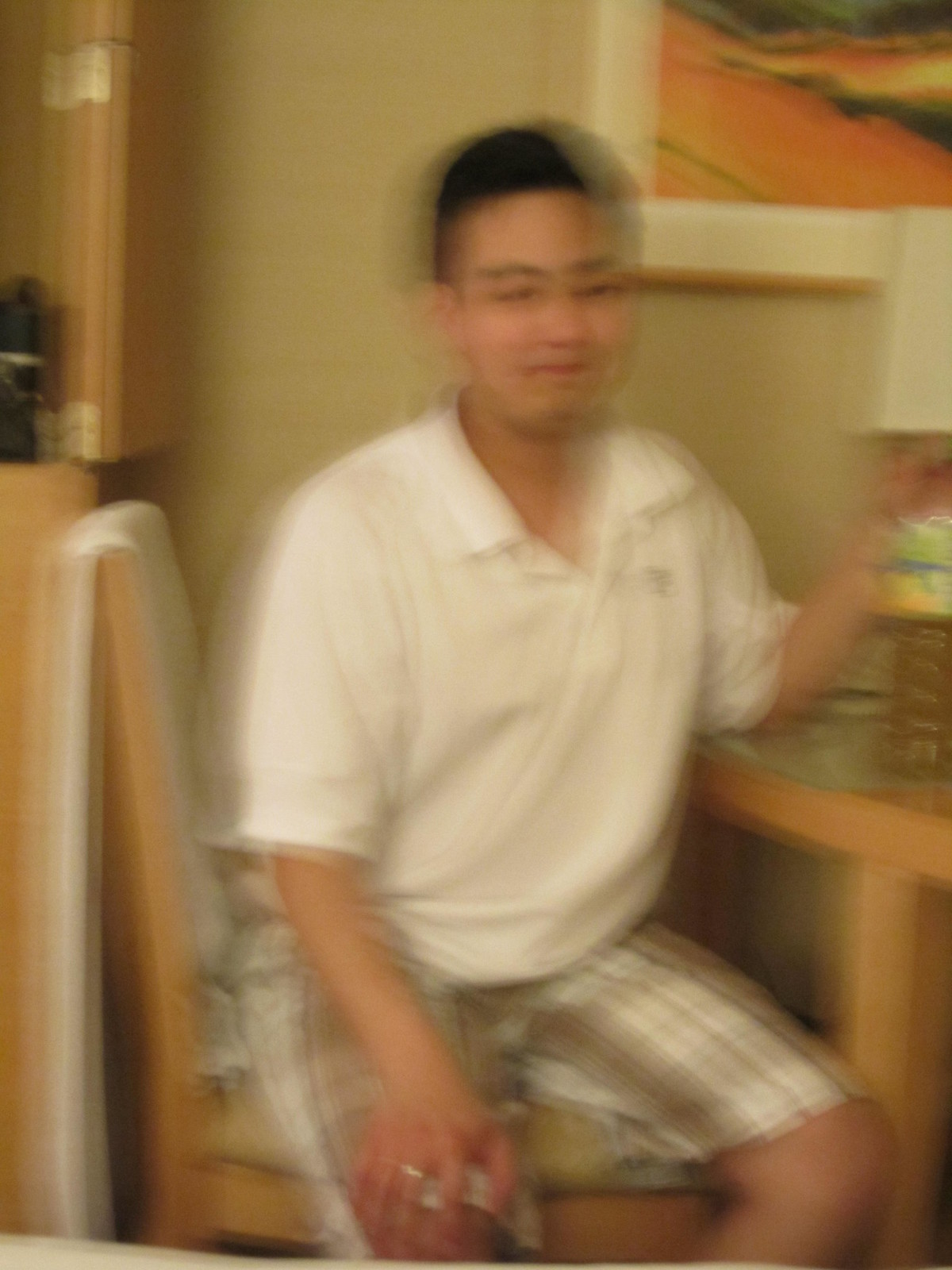The photograph is an extremely blurry color image, likely taken indoors at a dining or kitchen table. The setting includes a white wall adorned with a colorful painting that features orange and darker shapes, partially cut off by the edge of the image. The painting is encased in a simple rectangular wooden frame with a white canvas inside. The table in front of the wall is wooden and small, with only one of its legs visible, and it holds obscured objects that could be a small lamp and a dish of fruit.

Seated at the table is a man, who appears to be Asian, possibly Korean, characterized by his close-cropped, ear-length black hair. He is smiling and dressed in a white polo shirt with the top two buttons undone, paired with plaid tan and brown striped shorts. On his right hand, which is resting on his knee, he wears a ring that might be a wedding band, though it's indistinguishable due to the blurriness. The chair he occupies is wooden, tan-colored, and features a cushion with a white towel or tablecloth draped over its back. The entire composition is blurred, suggesting the camera was shaken during the capture.